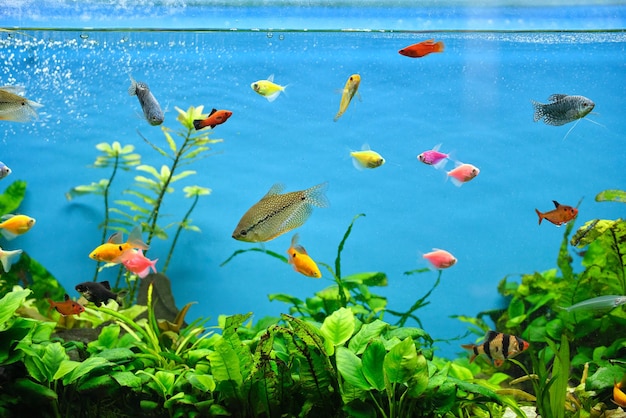In this vivid underwater photograph depicting the interior of a bustling aquarium, the scene is set against a vibrant blue backdrop studded with playful bubbles in the top left corner. The aquatic environment is teeming with life, showcasing around twenty fish in various colors and species. In the foreground, bright green leafy aquatic plants flourish, covering the bottom section and the bottom right corner of the frame.

Dominating the center of the image is a large, flat fish with a horizontal stripe running through its brownish-gray body, facing down to the left. Nearby, an orange fish with a black dot is positioned just beneath it. The bottom right corner features a striking black and orange striped fish moving from left to right, accompanied by another orange fish slightly above it. A gray fish, also heading left to right, sits above them in the top right corner.

The middle section of the photo highlights two vibrant fish: an orange one moving left just behind the gray fish, and a contrasting red fish swimming to the right. Above these, a brilliant red fighting fish adds a dynamic splash of color, paralleled by a yellowish fish ascending toward the water's surface. Close by, another yellow fish blends into the lively scene.

To the left of the gray fish, three more aquatic plants stand out, with a goldfish and another red fish swimming just beneath them. Additionally, nestled near the top of these plants is an orange fish with distinct black fins. The bottom left section of the background hosts more vegetation with yellow flowers, further populated by orange fish underneath.

The clear water of the aquarium and the glass top at the upper edge provide a pristine view into this captivating aquatic world, free of any text, inviting viewers to lose themselves in the tranquil beauty and vibrant diversity of underwater life.